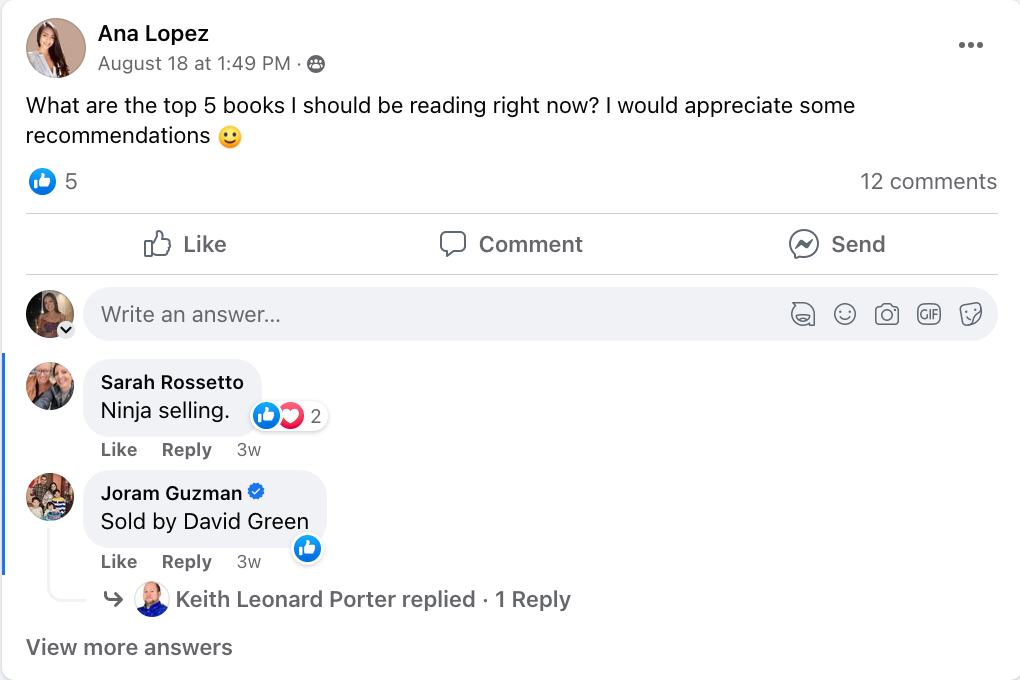In the image, a Facebook post by Anna Lopez is prominently displayed at the top. Anna, who has long black hair elegantly brushed over her shoulders, posted on August 18th at 1:49 PM asking for book recommendations: "What are the top five books I should be reading right now? I would appreciate some recommendations 😊." Her post has garnered five likes and twelve comments. Below her post, the options to like, comment, or send are clearly visible, along with a section showing the profile picture of the person currently viewing the post, complete with interactive icons for adding emojis, photos, GIFs, or files. Among the responses, notable mentions include Sarah Rossetto recommending "Ninja Selling" and Jerome Guzman suggesting "Sold" by David Green. One comment from Keith Leonard Porter also appears with an open reply, prompting viewers to "view more answers."